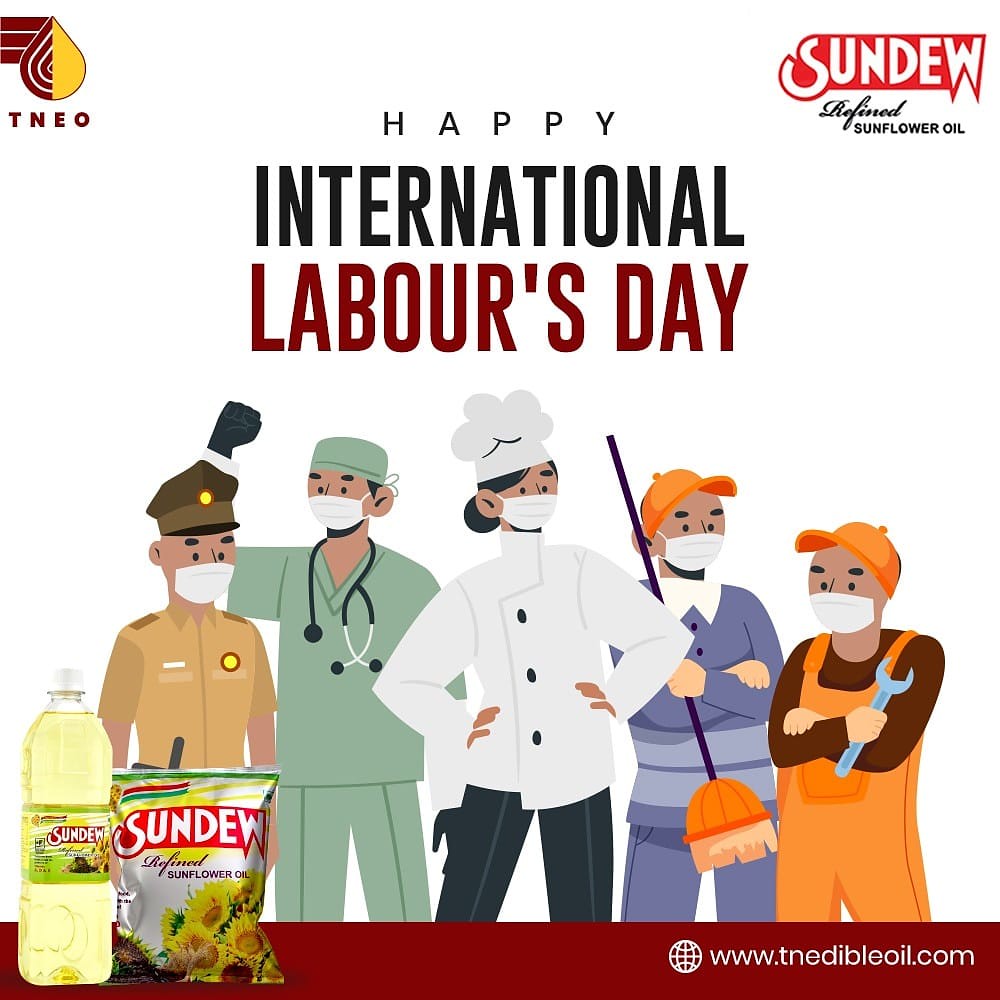This cartoonish advertisement, celebrating International Labor Day, prominently features the logos for TNEO and Sun Do Re-Defined Sunflower Oil. At the top left, there's a teardrop-shaped TNEO logo in red and yellow, while on the top right is the Sun Do Re-Defined Sunflower Oil logo. In large black and red text across the middle, it reads, "Happy International Labor Day." Below this message, there are five cartoon figures, each representing different careers and all wearing COVID masks: 

- A policeman or park ranger in a brown uniform with a walkie-talkie. 
- A nurse or doctor in light green scrubs, a stethoscope, and a raised fist. 
- A female chef in a white coat and hat, with dark pants.
- A janitor in purple clothing and an orange hat. 
- A handyman in orange coveralls holding a wrench.

At the bottom left, the Sun Do Oil container and a bag of Re-Defined Sunflower Oil are depicted, while the bottom right showcases the URL www.tnedibleoil.com in white font on a red rectangular background.